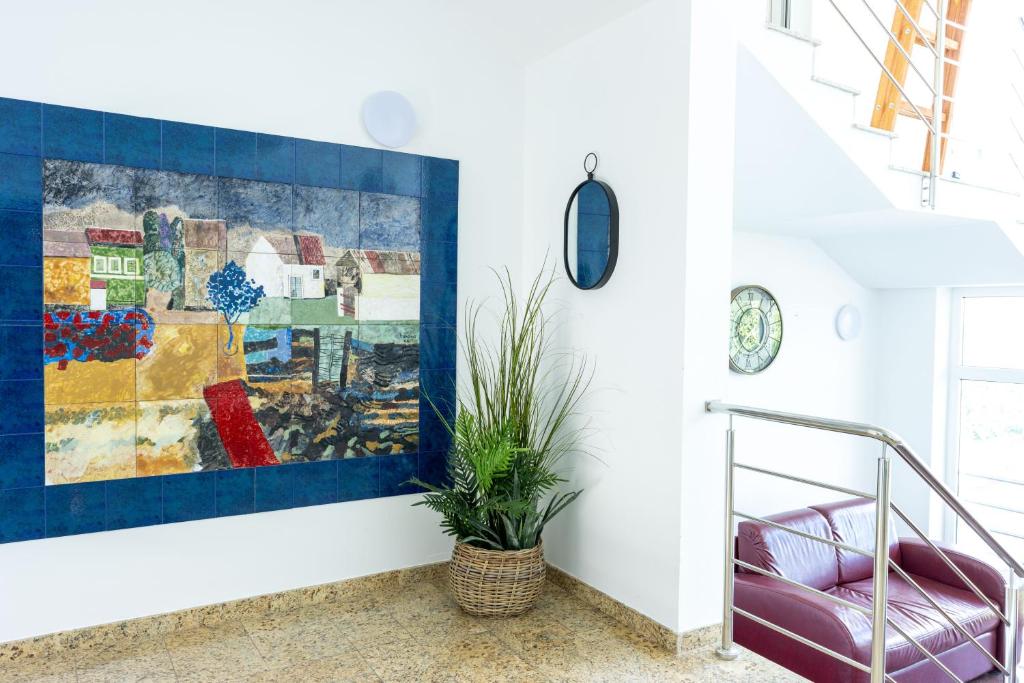This image depicts a bright, contemporary loft with a very abstract, eye-catching interior. Dominating the scene is an abstract painting on the left wall, featuring a colorful neighborhood rendered in a style reminiscent of puzzle pieces and bordered by a navy blue frame. The painting is rich with primary colors—red, blue, yellow, and green—creating a vivid focal point.

Adjacent to the painting is an artificial plant, thriving in a wooden basket. The plant features wispy, long grass blades complemented by thicker ferns at the base. Nearby, a mirror hangs on the wall, adding a sense of depth to the space.

The loft’s white walls contrast with mustard-colored marble tiling on the floor. On a slightly lower level, a red sofa chair stands near the entryway, appearing purplish under the bright daylight. Above this area, a green clock adorns the wall. A wooden ladder leans against the stairway, suggesting a three-story layout with two visible sets of stairs. The room's modern charm is accentuated by its openness and the play of light, emphasizing its abstract and dynamic design.